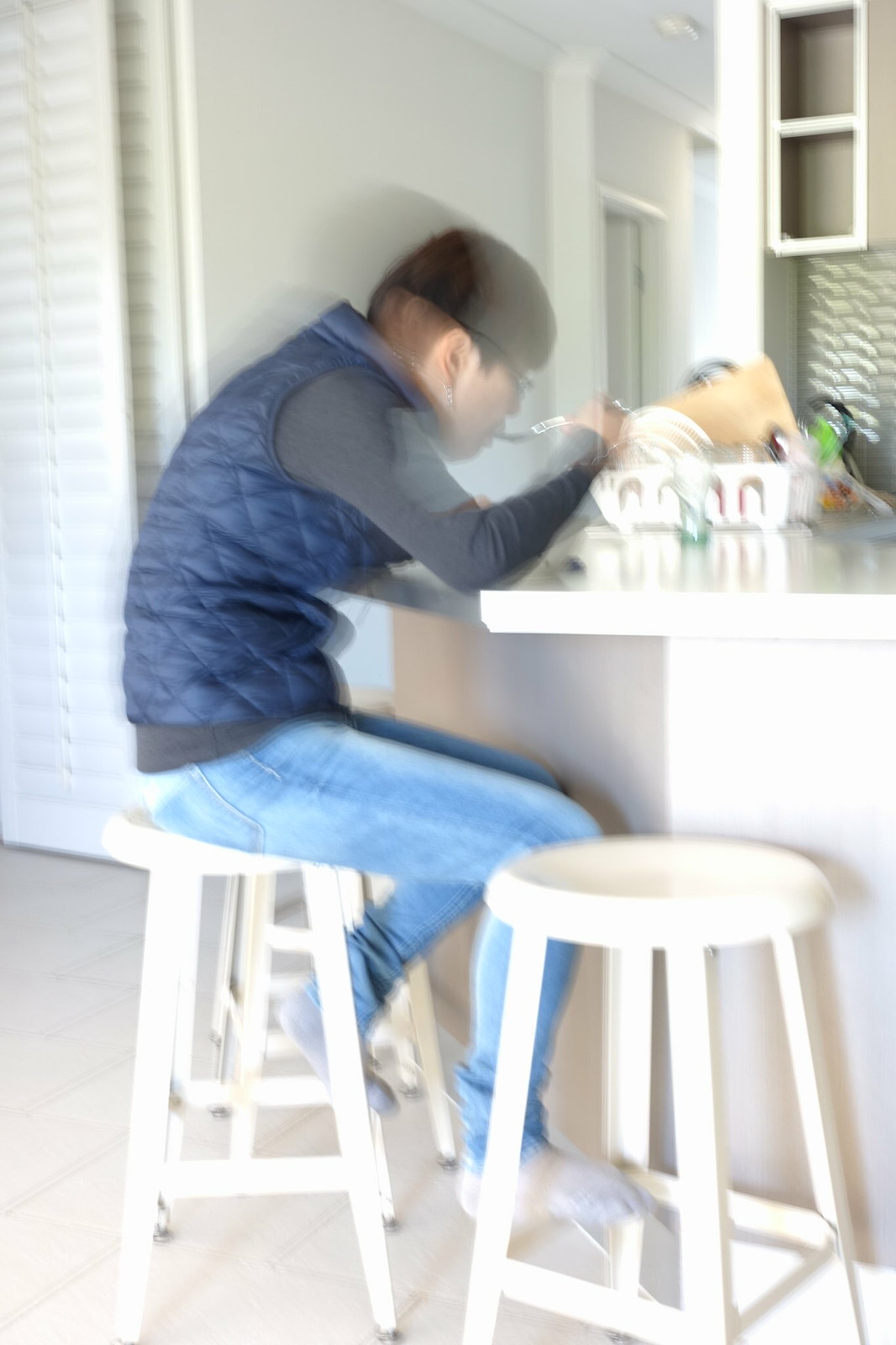The image depicts a man seated at a white kitchen counter, which occupies the center of the photo. He is perched on the second of two white metal barstools, with his right foot resting on the adjacent stool and his left foot on the stool he is seated on. The man is wearing blue jeans, socks, a gray long-sleeve shirt, and a blue vest. His black hair is cropped short in the back but longer on top, and he is wearing glasses. He appears to be eating, holding a spoon to his mouth with his right hand, and his right arm is bent at the elbow. 

The setting includes various white elements: a white wooden floor, a white counter, and walls, contributing to a bright, monochromatic ambiance. Behind the man is a white draining board containing dishes and a brown cutting board, which is partially blurred due to the photo's slight double exposure effect. The backdrop also features a white slatted window with blinds, a small white cabinet with brown rectangles, and a silver backsplash area beneath it. The entirety of the setting emphasizes a clean, minimalistic kitchen environment.